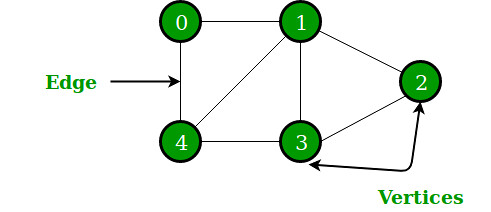The diagram depicted in the image appears to have been created digitally. On the left side, the word "Edge" is displayed in green text, with a black arrow pointing towards a thin black line. At the top end of this line, there is a green circle containing the number "0," and at the bottom end, there is another green circle with the number "4."

Two lines extend horizontally to the right from these circles. In the upper right corner is a green circle with the number "1," and directly below it, another green circle with the number "3." A diagonal line connects the circles labeled "1" and "4," forming part of a square shape within the diagram. 

From the circle labeled "1" and the circle labeled "3," additional lines extend inward but meet at an intermediary circle labeled "2," creating a more complex intersection.

In the bottom right corner, the word "Vertices" is noted, with two black arrows extending from it. One arrow points towards the circle labeled "3," and the other points towards the circle labeled "2."